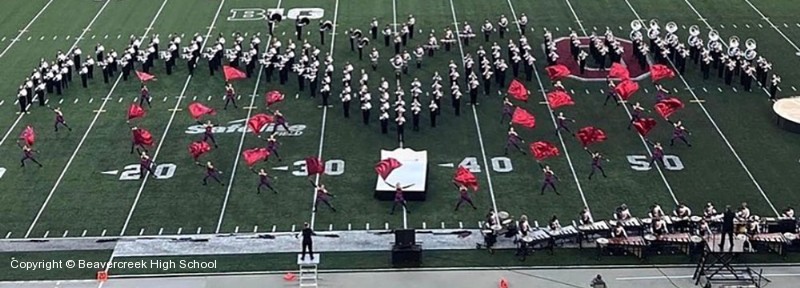The photograph captures halftime at a football game in an outdoor stadium, likely Beaver Creek High School, as indicated by the copyright notice in the bottom left corner. The image shows the green astroturf field marked with the 20, 30, 40, and 50-yard lines. At the center of the image, a marching band is arranged in a wave formation resembling a seagull, with their predominantly white uniforms featuring dark bottoms. The formation peaks between the 30 and 40-yard lines, then curves downward towards the sidelines. Beneath the band’s wingspan, roughly ten people are holding red triangular flags, and along the sidelines, there are onlookers, including individuals possibly filming the performance and others gathered near tables. At the very bottom of the image, two men are positioned on podiums, directing the band. The overall scene combines the structured artistry of the marching band with the bustling activity typical of a halftime show.